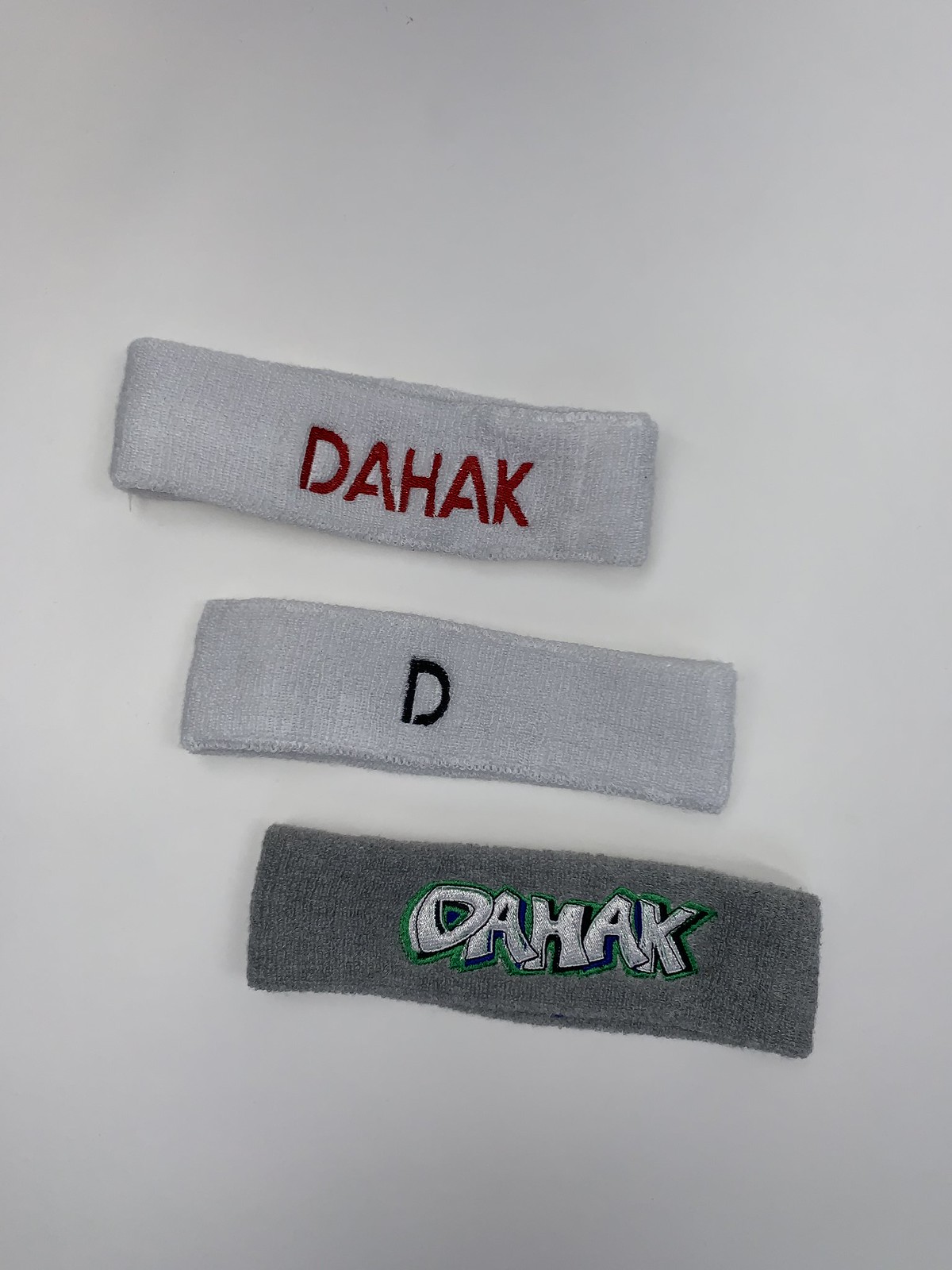The color photograph showcases three distinct sweatbands, centrally positioned against a primarily white background with subtle gray shadows. Each sweatband appears to be made of stretchy elastic cloth and is horizontally oriented, slightly tilted, and stacked vertically with space separating them. The topmost sweatband is light gray and features the red embroidered capital letters "D-A-H-A-K," though it appears to have some dirt or soil on it. The middle sweatband is also light gray and prominently displays a single black capital letter "D" in the center. The bottom sweatband, in dark gray, is adorned with "D-A-H-A-K" in a striking silver graffiti-style font, bordered by green and blue accents around the edges.